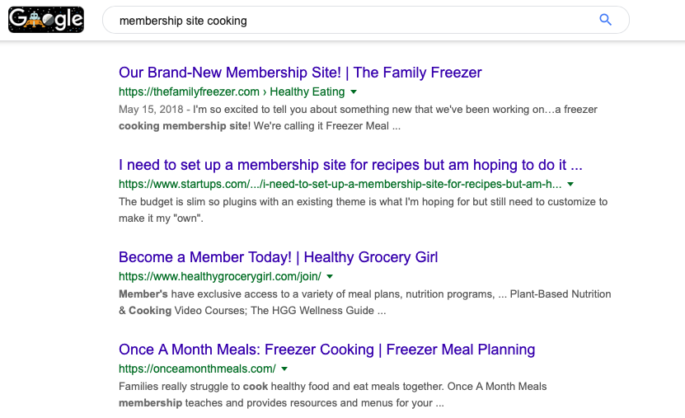This image showcases a Google search for "membership site cooking." The search results present four entries, each detailed as follows:

1. **Our Brand New Membership Site: The Family Freezer** 
   - URL: [https://thefamilyfreezer.com](https://thefamilyfreezer.com) - Healthy Eating
   - Date: May 15, 2018
   - Description: "I'm so excited to tell you about something new that we've been working on, a freezer cooking membership site. We're calling it Freezer Meal."

2. **I Need to Set Up a Membership Site for Recipes**
   - URL: [https://www.startups.com](https://www.startups.com) 
   - Description: "I need to set up a membership site for recipes, but the budget is slim, so plugins with an existing theme is what I'm hoping for, but still need to customize to make it my own."

3. **Become a Member Today: Healthy Grocery Girl**
   - URL: [https://www.healthygrocerygirl.com/join](https://www.healthygrocerygirl.com/join)
   - Description: "Members have exclusive access to a variety of meal plans, nutrition programs, plant-based nutrition and cooking video courses, the HGG Wellness Guide."

4. **Once a Month Meals: Freezer Cooking, Freezer Meal Planning**
   - URL: [https://onceamonthemeals.com](https://onceamonthemeals.com)
   - Description: "Families really struggle to cook healthy food and meals together. Once a Month Meals membership teaches and provides resources and menus for your family."

Each result includes a purple-tinted heading, a green URL, and additional descriptive text in gray, providing a comprehensive overview of various cooking membership sites.